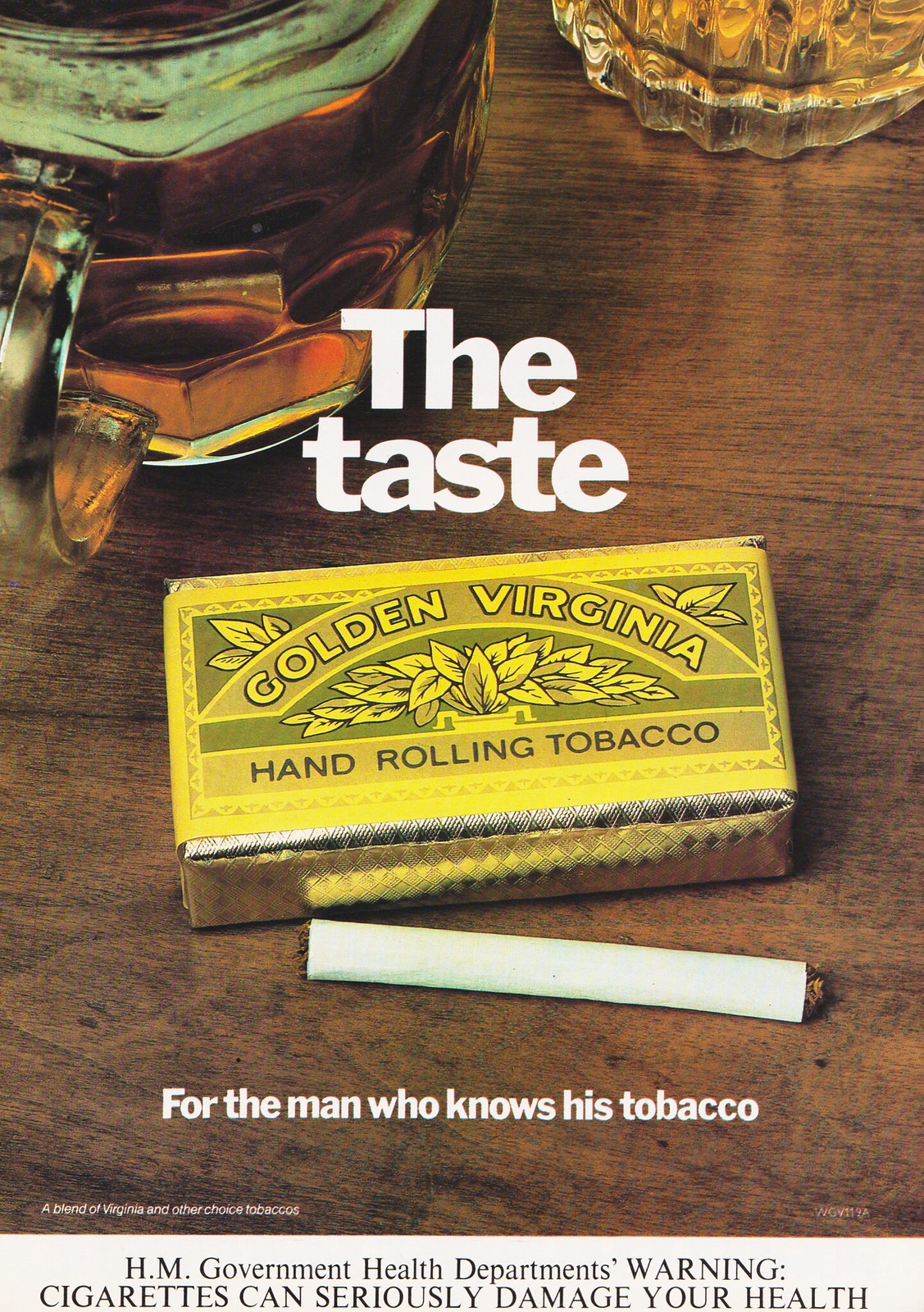The vertical rectangular image is an advertisement for Golden Virginia Hand Rolling Tobacco, prominently displayed on a beautifully grained wooden table. In the middle of the image is a small yellow box adorned with dark green detailing and leaf illustrations, labeled "Golden Virginia Hand Rolling Tobacco." In front of the box lies a hand-rolled cigarette with tobacco visibly protruding from each end. The top of the image features the bold white text "The Taste," accompanied by the subtext "For the man who knows his tobacco" in smaller letters underneath. In the top left corner, a mug filled with amber beer can be seen, while a smaller glass of an alcoholic beverage occupies the top right corner. At the bottom, the English government's health warning is clearly visible, stating, "Cigarettes can seriously damage your health."